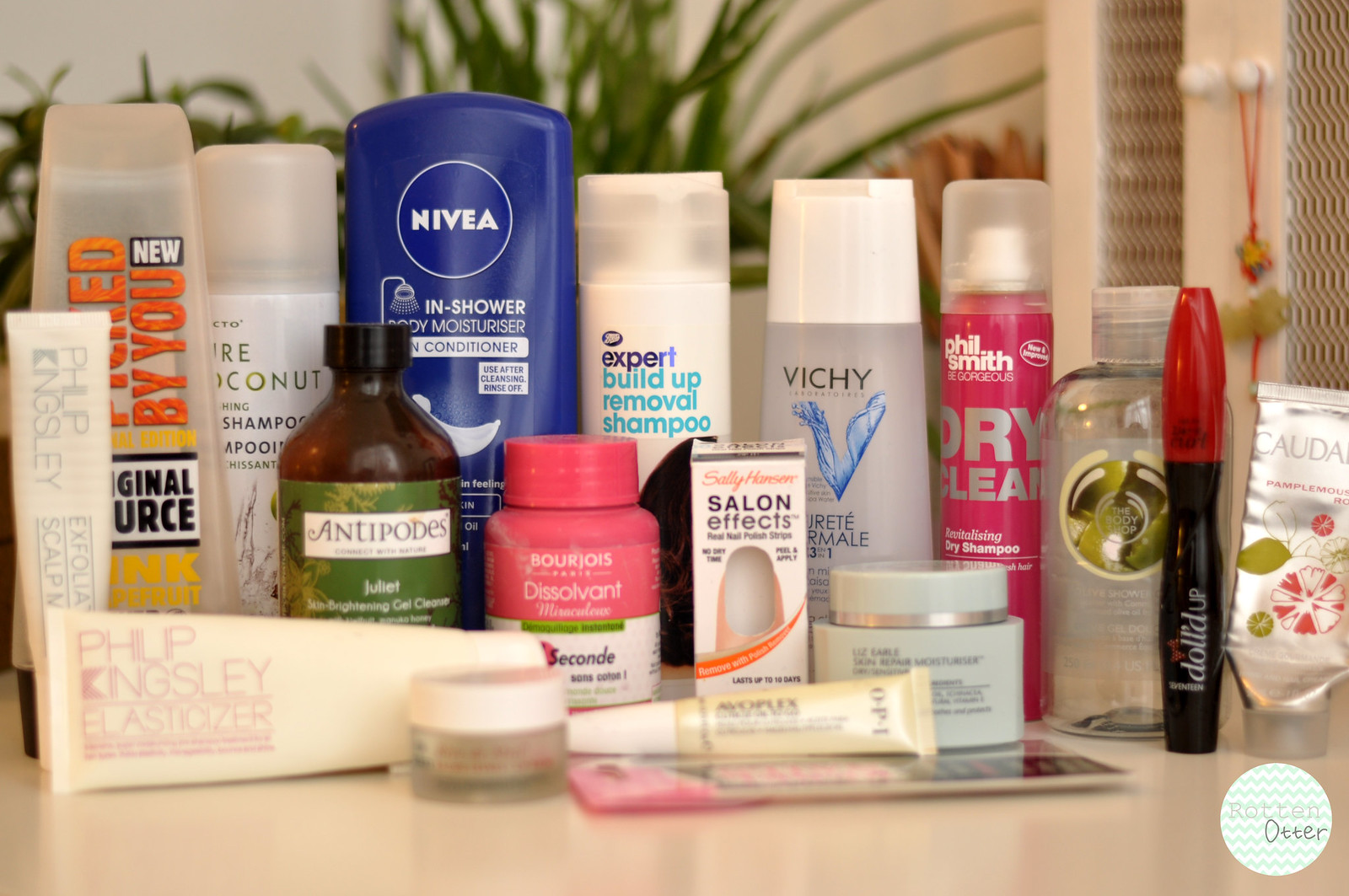This well-lit photograph captures an assortment of approximately 20 toiletry and beauty items neatly arranged on a pristine white counter, likely in a bathroom setting. A plant with dark green leaves, slightly out of focus, adds a touch of nature in the background. To the right, the blurred silhouette of cabinet doors hints at a storage area.

On the far left, there's a tube labeled "Philip Kingsley Exfoliate Scalp" with part of the text obscured. Adjacent to it is another "Philip Kingsley" product, an "Elasticizer" tube. Behind them, a couple of bottles are identifiable as shampoos. Next in line, a blue bottle features the label "Nivea In-Shower Body Moisturizer Skin Conditioner." In front of it, a dark bottle marked "Antipodes Juliette Skin Brightening Gel Cleanser" stands prominently.

Toward the front of the assembly, a smaller container and a pink bottle labeled "Bourjois" catch the eye. Another bottle of shampoo, nail polish strips, and various other partially readable bottles, likely including more shampoo, dry shampoo, lotion, and a container of mascara, complete the arrangement.

The composition of the items presents a harmonious blend of textures and colors, creating an inviting and organized display of self-care essentials.